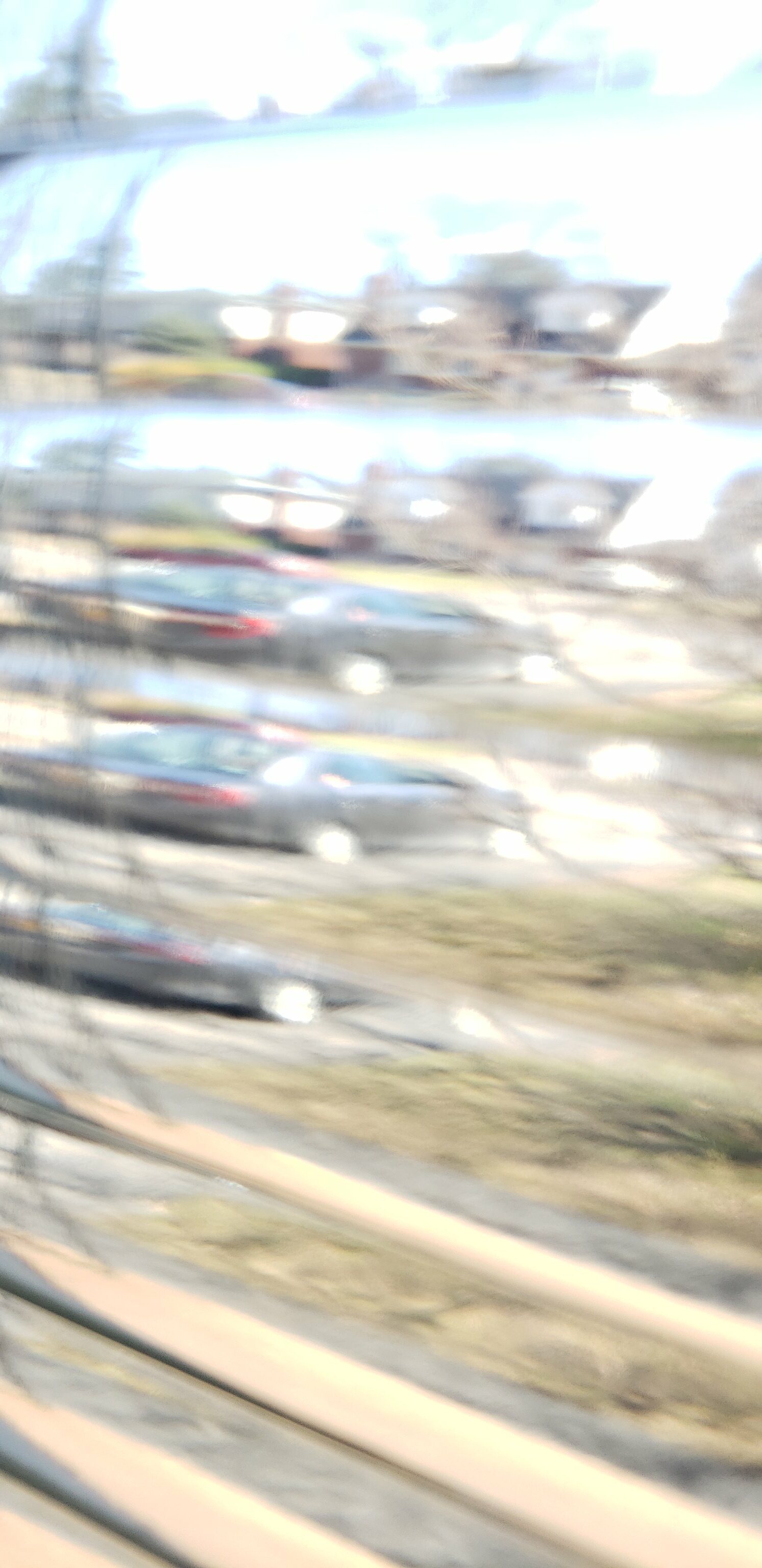The image features a gray parked car viewed through partially opened white blinds. The scene includes a green outdoor space, and another home is visible across the street. The top portion of the image provides a clear, unobstructed view, revealing a bright blue daytime sky. As the gaze moves downward, the white blinds become more prominent, suggesting they are cracked open rather than lifted.